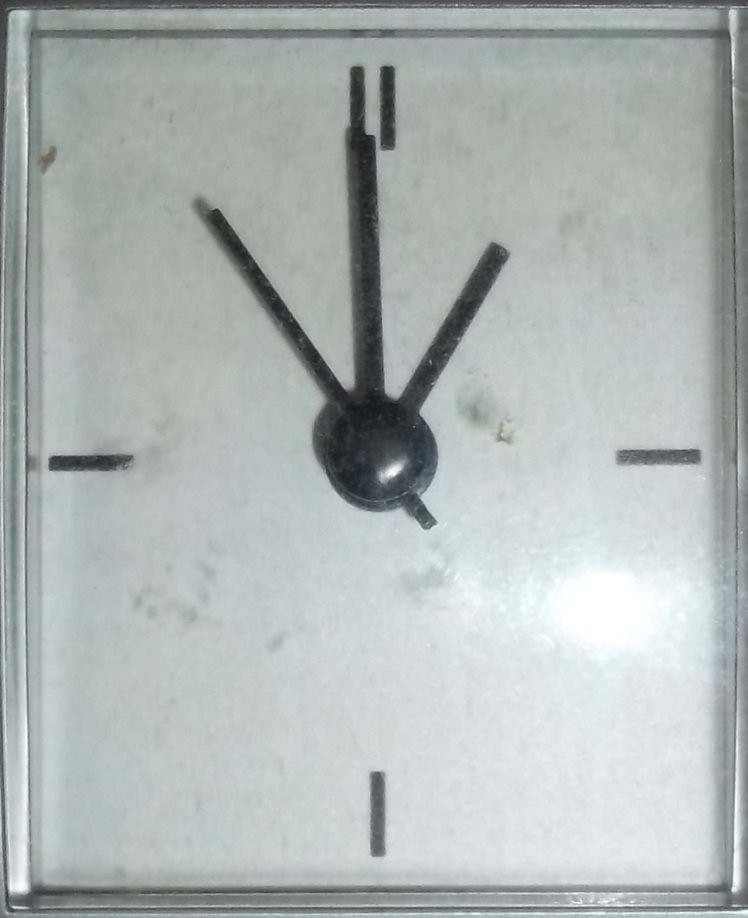The image showcases a uniquely designed rectangular clock with a sleek silver frame. The clock face features a predominantly white background with subtle gray splotches, giving it a marbled effect. Unlike traditional clocks, this one lacks numerical markings. Instead, the positions where numbers would usually appear are indicated by minimalist lines: two small parallel lines resembling the numeral "11" at the 12 o'clock position, a single horizontal line at the 3 o'clock position, another horizontal line at the 9 o'clock position, and a vertical line at the 6 o'clock position. The clock is equipped with hour, minute, and second hands, currently indicating the time as 1:00. In the right-side region of the clock face, just below the 3 o'clock marker, there is a noticeable glare caused by the camera flash reflecting off the surface.